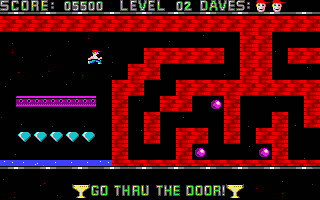The image showcases a vintage-style video game screen featuring a maze. The centerpiece of the visual is a small character dressed in a red hat, blue jeans, and a brown shirt, who appears to be navigating the red maze. The maze is set against a black background, contributing to a stark contrast that highlights the navigational paths. At the bottom of the screen, green text reading "Go through the door!" is prominently displayed, flanked by yellow trophy icons on either side, against a black backdrop. Above this text is a horizontal gray-striped line, followed by a blue-striped line on the left that leads to five blue diamonds and a purple platform. Additionally, three purple balls are positioned at the bottom of the maze, adding to the maze's complexity. The top section of the screen provides game status information, reading "Score: ... 05500 Level 02" followed by "Dave's," accompanied by two Dave icons. This text is also in green, maintaining consistency with the instructional text below.